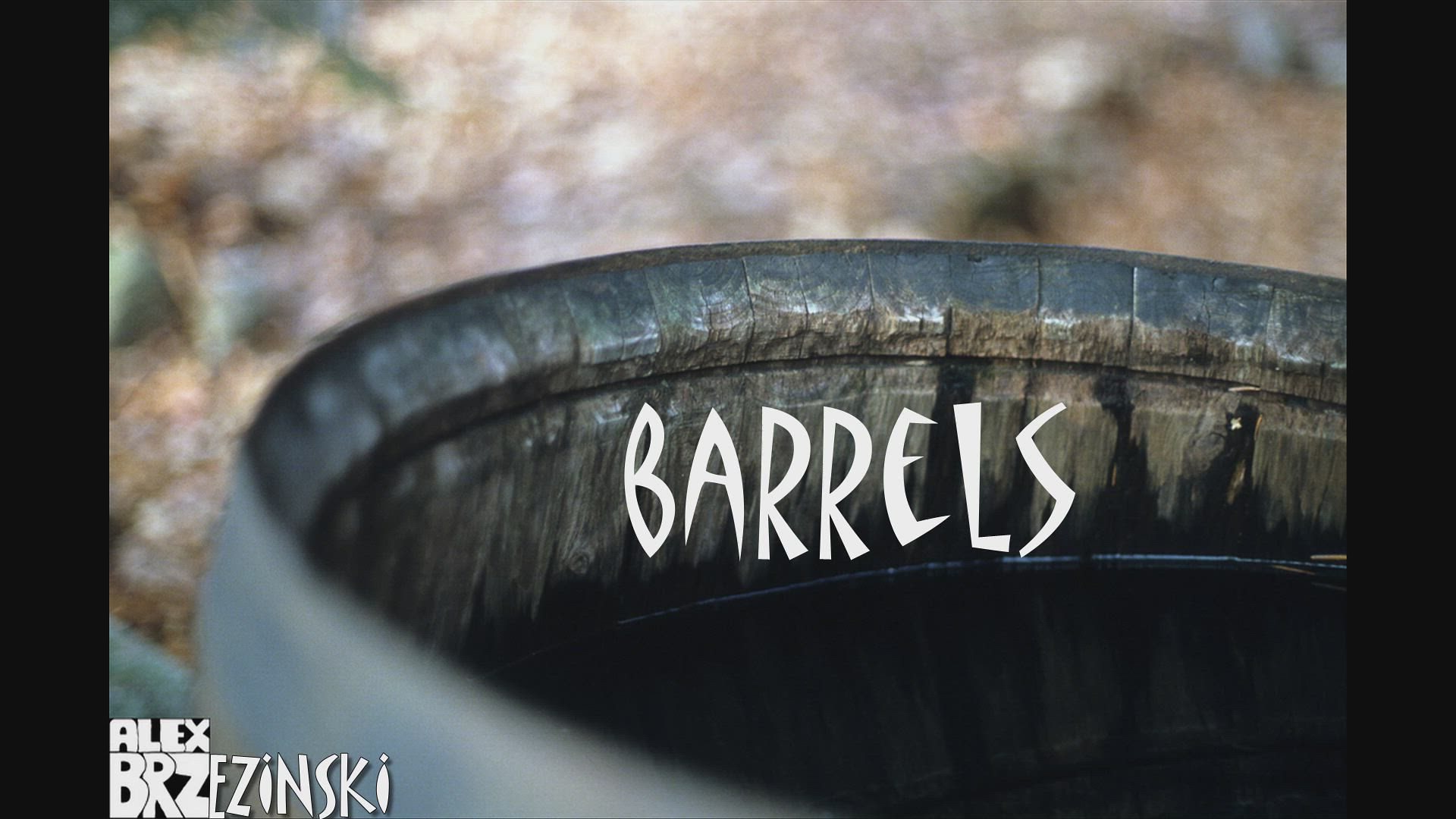The image captures a close-up of the weathered, bluish-gray top edge of an old, possibly handmade wooden barrel, showcasing its vertical wooden slats and metal bands that hold them together. The inside of the barrel is a rich brown, suggesting it may be filled with liquid up to about four inches from the top. In the center of the barrel's upper rim, "BARRELS" is prominently displayed in stylized, all-caps white text, and in the lower left corner, the name "Alex Brzezinski" appears in similar print. The background is blurred, giving a faint impression of dead leaves, indicating that the scene is outdoors during the day. The barrel's worn appearance and subtle details, such as its beautiful bluish patina, add to its rustic charm.